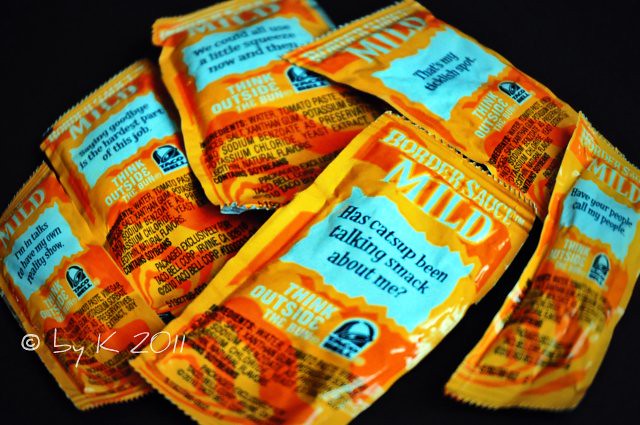The image depicts six Taco Bell Border Sauce Mild packets arranged in a somewhat circular pile, spanning from the top to the bottom and left to right of a landscape-oriented photo. Each packet features a gradation of orange, ranging from a lighter shade to a darker one, with the text predominantly in black and white. The top part of the packet reads "Border Sauce Mild" in white typography. Below, in a white conversation bubble, are humorous sayings written in black. The most prominent packet facing the viewer humorously asks, "Has ketchup been talking smack about me?" Other legible packets bear phrases like, "I'm in talks to have my own reality show," "Saying goodbye is the hardest part of this job," "We could all use a little squeeze now and then," "That's my ticklish spot," and "Have your people call my people." The iconic Taco Bell logo in black and white is positioned towards the bottom of each packet. The ingredients are also displayed on the front, maintaining Taco Bell’s characteristic quirky style.